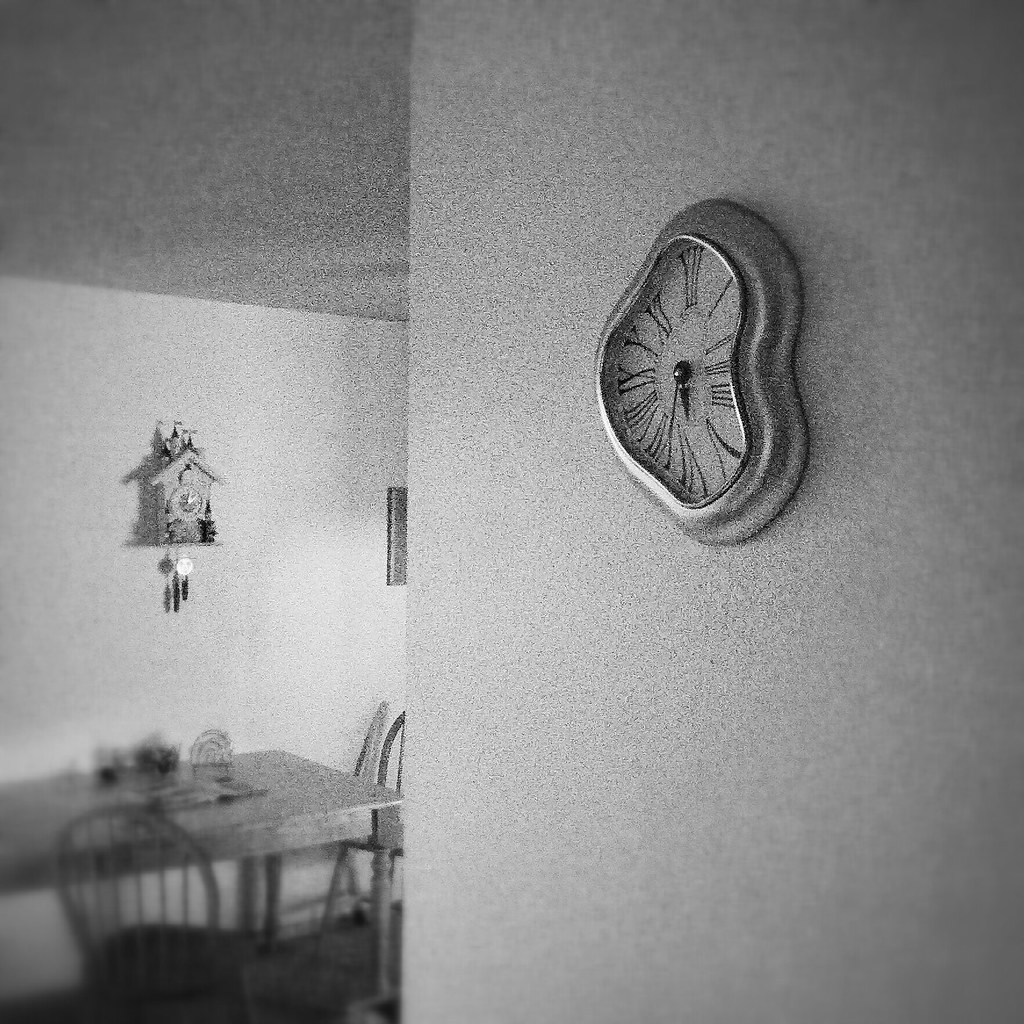This intricately detailed charcoal drawing depicts an interior scene dominated by two contrasting clocks. In the foreground, a gray, shadowed wall features a prominently misfigured clock, reminiscent of Salvador Dalí's melting timepieces. This distorted clock, marked with Roman numerals, shows the time as approximately 5:33. 

Beyond the wall, part of a room is visible, featuring a traditional cuckoo clock hanging on the far wall, its hands pointing to around 2:05. The room contains a simple wooden table set with two chairs, and several indistinct items rest on the table's surface. A partially visible picture frame is obscured by the foreground wall.

The meticulous shading and attention to detail in the drawing highlight the surreal contrast between the melted clock in the foreground and the seemingly functional cuckoo clock in the background, creating a thought-provoking juxtaposition.